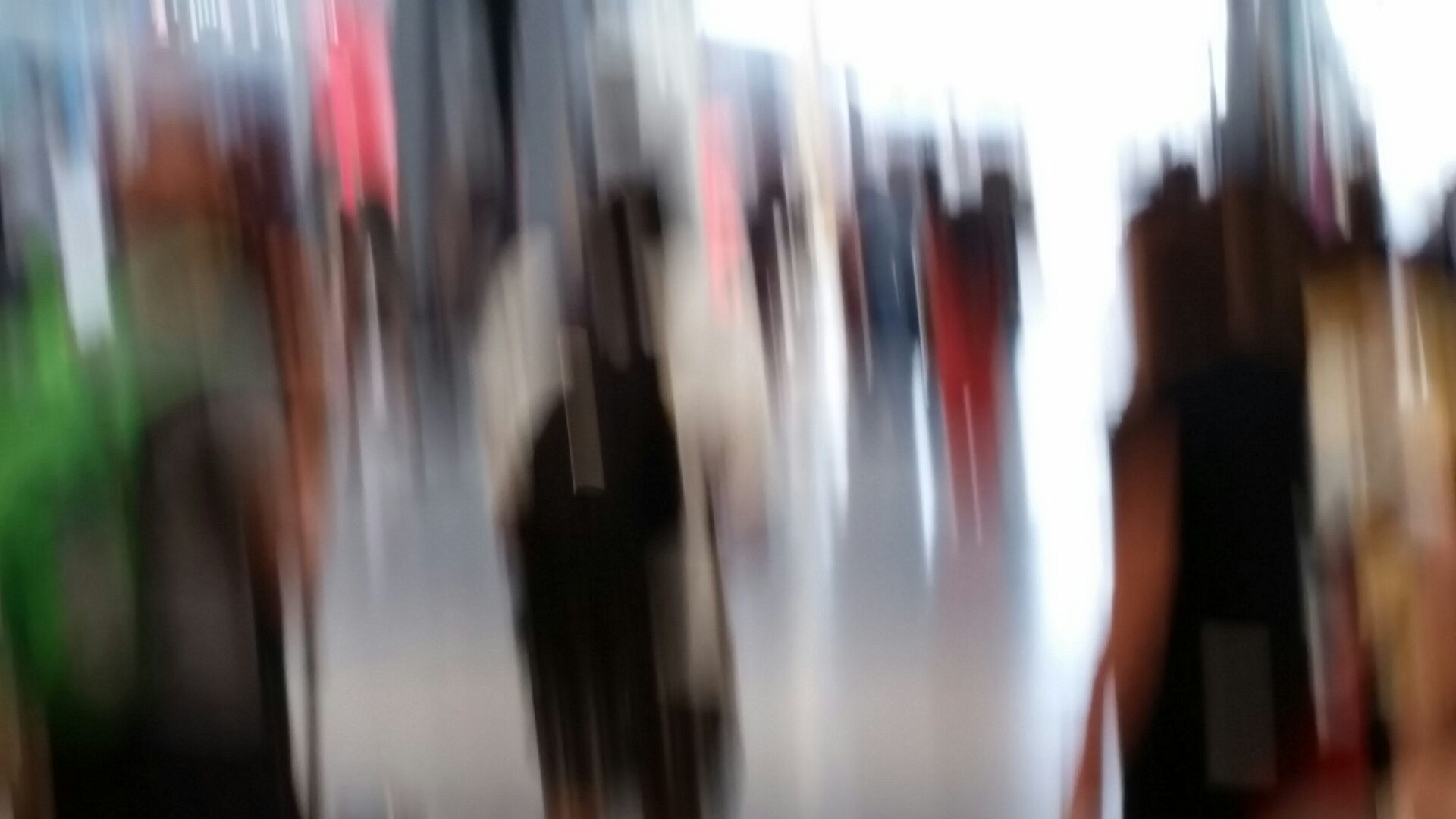A highly blurry photo captures a busy shopping area or plaza, likely taken accidentally from hip height, suggesting the photographer was retrieving their phone from a pocket or bag when the picture was snapped. The image shows approximately a dozen indistinguishable figures, their forms obscured by the motion blur. Bright natural daylight floods the scene, indicating the photo was taken during daytime, but the details of the setting and individuals remain vague due to the lack of focus.